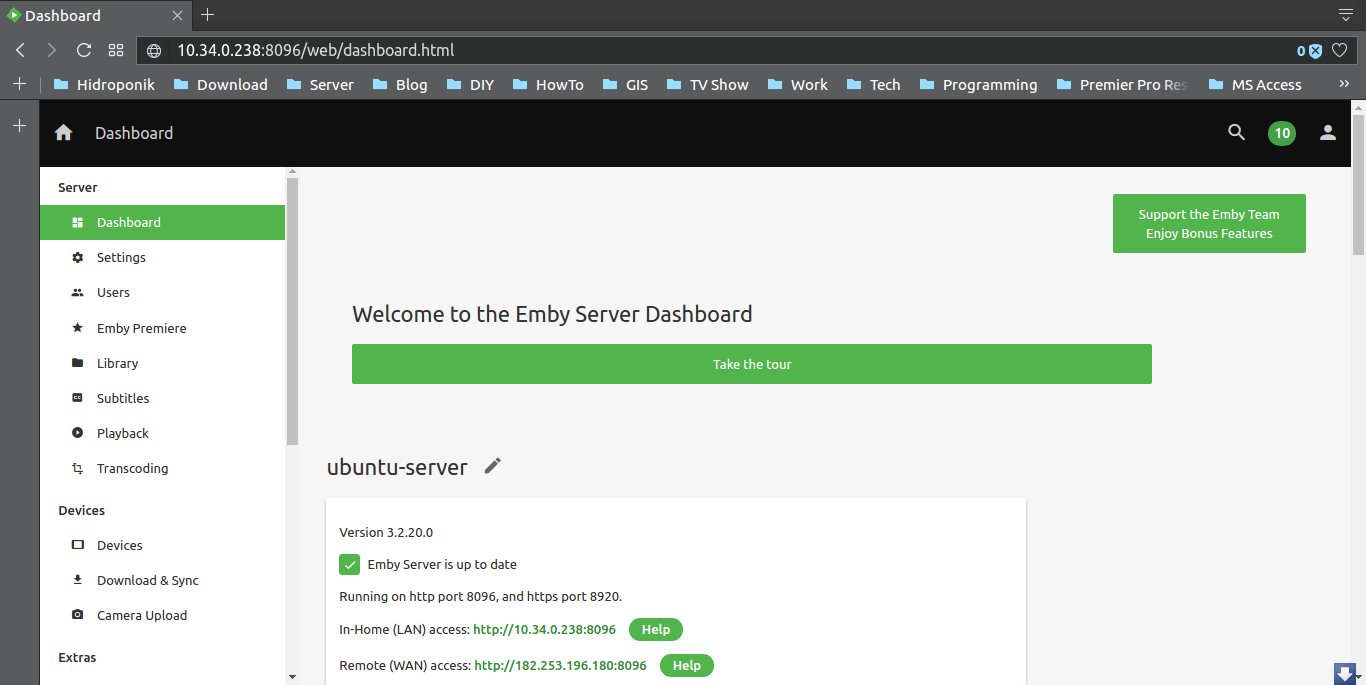In the provided image, the main focus is a website interface displaying a server dashboard. 

**Top Section**:
- Top-left corner: The tab is labeled "Dashboard."
- Below the tab: The URL of the site is displayed.

**Left Sidebar**:
- Features a series of tabs and categories, each identified with a light blue icon and white text:
  - Dashboard (default tab)
  - Settings
  - Users
  - MB Premiere
  - Library
  - Subtitles
  - Playback
  - Transcoding
  - Devices
  - Downloads
  - Sync
  - Camera Upload
  - Extra

**Dashboard Interface**:
- Below the URL: A black background stripe containing the dashboard label, flanked by icons:
  - Left: Home icon
  - Center-left: Search icon
  - Center-right: Blue circle with the number “10”
  - Right: Profile icon
  
**Main Content Area**:
- Header: Reads "Welcome to the MB Server Dashboard."
- Two green rectangles:
  - Smaller one: "Support the MB team, enjoy bonus features."
  - Larger one lies directly below.

**Footer**:
- Bottom of the screen: "UBUNTU server" followed by three or four lines of text referring presumably to server details.

**Background**:
- Right side: Light gray background highlights the contrast with the main dashboard content.

This detailed description meticulously captures each element and feature for a comprehensive understanding of the webpage layout.